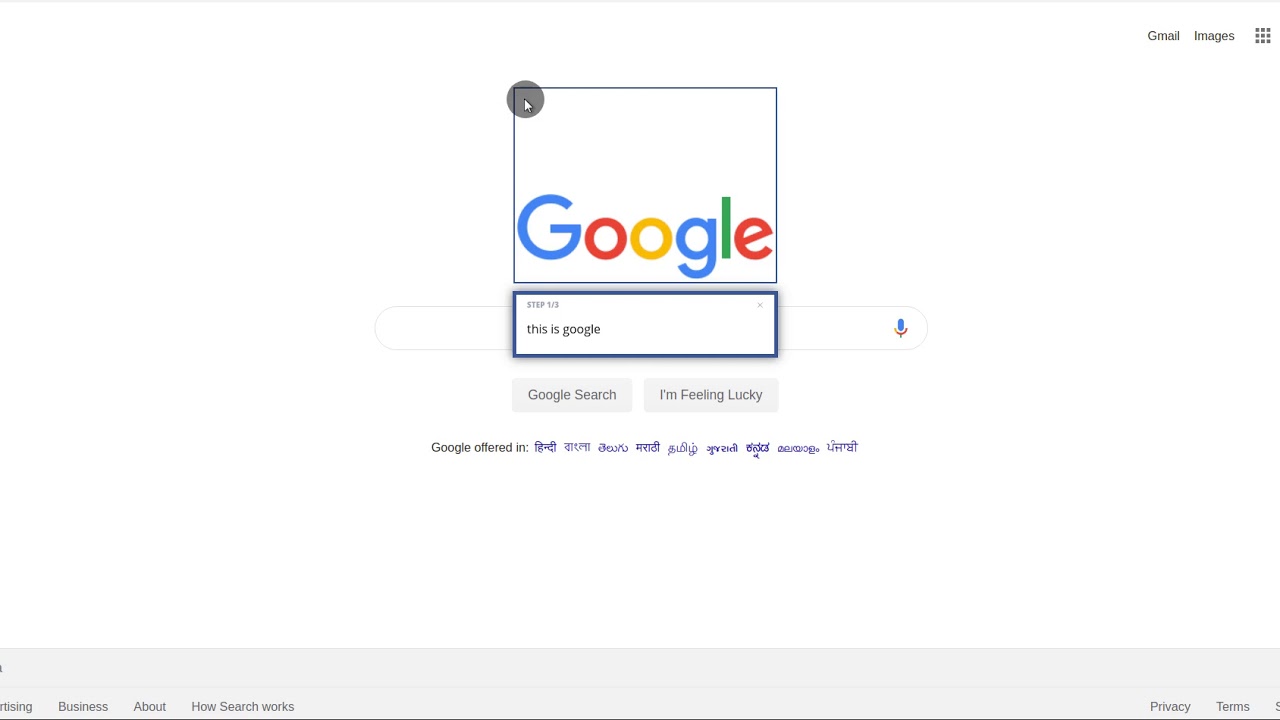This image is a detailed screenshot of a Google search page. At the top, the iconic Google logo is prominently displayed within a rectangular box. The logo features a blue uppercase "G," followed by a red lowercase "o," a vibrant yellow lowercase "o," a blue lowercase "g," a green lowercase "l," and concludes with a red lowercase "e."

Beneath the logo, there is an empty search box indicating "step one of three." The phrase "this is Google" is typed into the search field. Adjacent to the search box on the right is a microphone icon, suggesting the availability of voice search.

Below the search box, there are two light gray buttons. The left button is labeled "Google Search," and the right button reads "I'm Feeling Lucky."

Further down the page, small text in light gray notifies users about the available languages in which Google is offered, featuring what appears to be Hindi script, among others. A faint gray bar beneath this text has partly obscured words that might include "advertising."

To the right of the partly cut-off text, clickable links are sequentially listed as follows: "Business," "About," and "How Search Works." On the far right side of the page, additional links for "Privacy" and "Terms" are also visible.